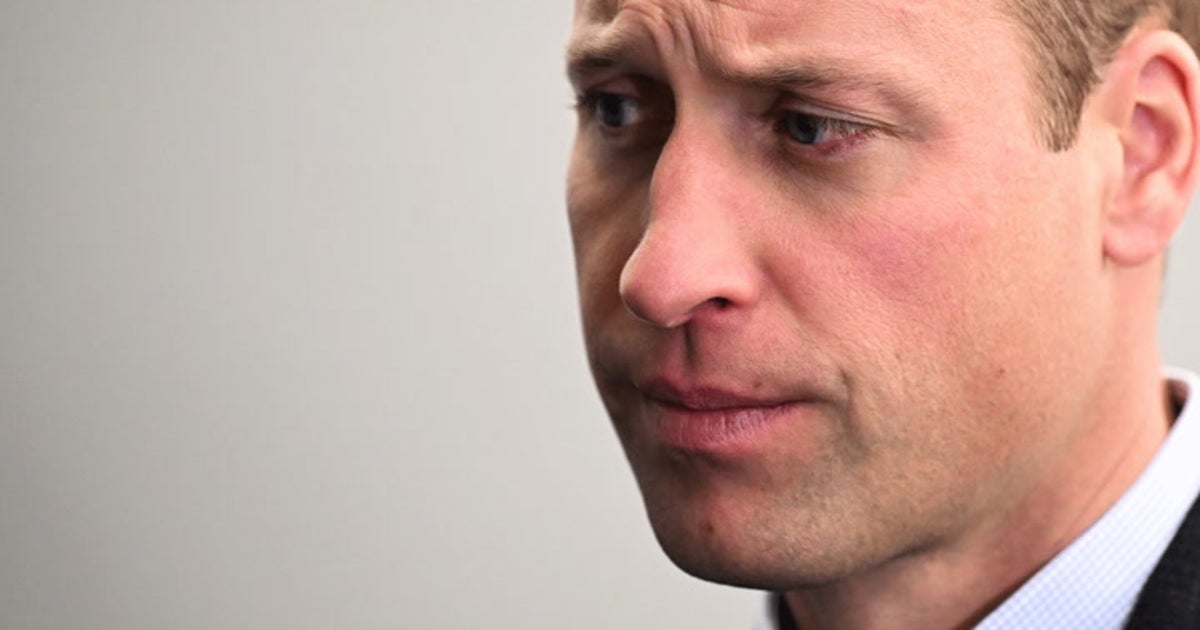This detailed color photograph offers an intimate close-up of Prince William's face in profile, primarily showcasing the left side of his face with a slight glimpse of the right. His short brown hair is visible near his left ear, and his furrowed brow and tight-lipped expression, which suggests a frown or a slight sense of upset, dominate his features. The background is a blank, white wall, adding a stark contrast to the image. He is dressed in a white shirt with a tiny blue-checked collar, just peeking out, and the upper part of a dark-colored, likely navy blue or black blazer is visible towards the bottom right of the image. The photograph frames him from just above the eyebrows to around his chin, and his focused gaze is directed towards the left.